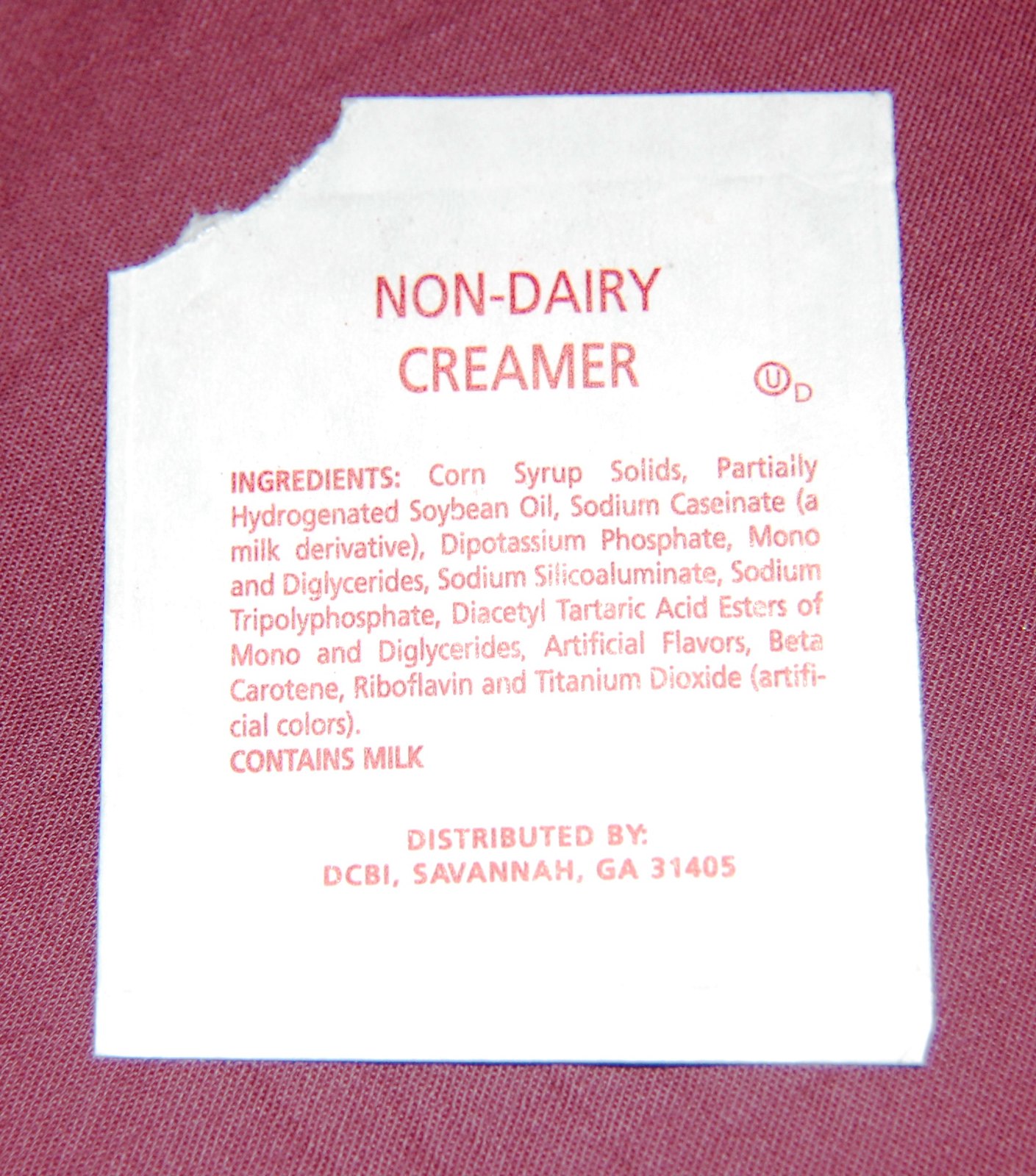This image depicts an opened packet of non-dairy creamer, likely showing the back of the packet. The upper left-hand corner is visibly torn open. The packet rests on a red background, which appears to be either a table or a cloth material.

The visible list of ingredients includes: 
- Corn syrup solids
- Partially hydrogenated soybean oil
- Sodium caseinate, a milk derivative
- Dipotassium phosphate
- Mono and diglycerides
- Sodium silico aluminate
- Sodium triphosphate
- Diacetyl tartaric acid esters of mono and diglycerides
- Artificial flavors
- Beta carotene
- Riboflavin
- Titanium dioxide, an artificial color

Furthermore, the packet specifies that it contains milk. At the bottom, the packet notes that it is distributed by DCBI, Savannah, Georgia 31405.